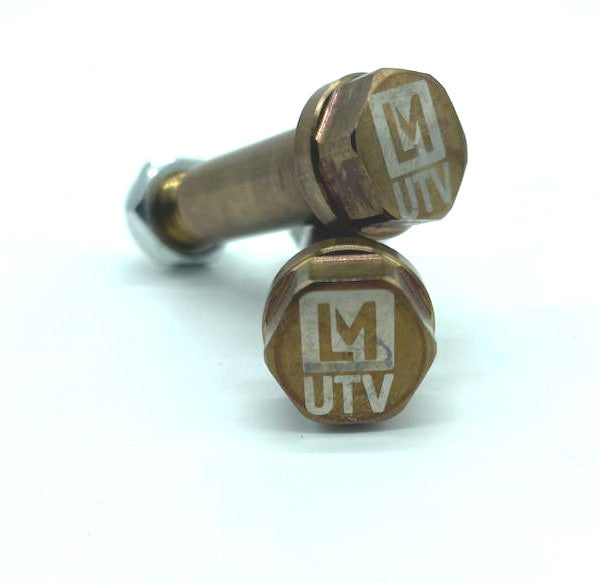The image showcases two gold-colored metal bolts with hexagon-shaped heads, although the corners of these heads are rounded. Both bolts display the brand "LMUTV" on their tops, printed in white letters. One bolt is leaning against the other, and the leaned bolt's brand-marked top faces the top right of the image. Each bolt is accompanied by a washer of the same golden hue snug against the end. Notably, the bottom end of the top bolt is equipped with a silver nut, contrasting with the otherwise golden color.